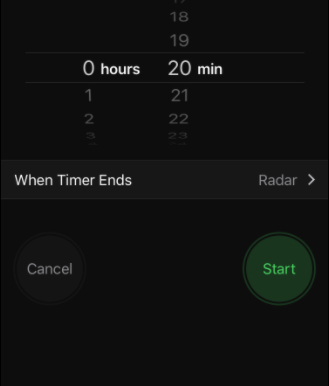A detailed descriptive caption for the image could be:

"The screenshot captures a sophisticated digital timer interface designed to track intervals with precision. The background is uniformly black, providing a stark contrast for the bright white numbers that denote time. These numbers are arranged in a vertical, rotating format, enabling users to set specific durations easily. The time increments are meticulously displayed, with the minutes ranging from 0 to 59 and the hours from 0 to 12. Central to the interface, a green 'Start' button enables the commencement of the countdown, while a black 'Cancel' button with grey lettering allows for termination. The word 'Radar' is prominently displayed in light gray text, tagged to the side of the interface, possibly indicating an additional feature or functionality. The overall design is sleek and user-friendly, ideal for precise timekeeping tasks."